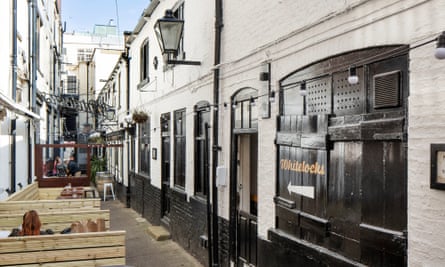The image captures a narrow, modern alleyway nestled between two white buildings with black trim. The left building features a distinctive upward-pointing arrow on its façade, while the right building has black trim at the bottom and a black square light fixture with transparent glass. Across from the right building, wooden sitting areas made of timber provide a place to rest, and a woman can be seen sitting there. Farther down the alley, there's a white chair and additional people sitting in the distance. The sky overhead is a light blue, adding to the calm and inviting atmosphere of the scene.